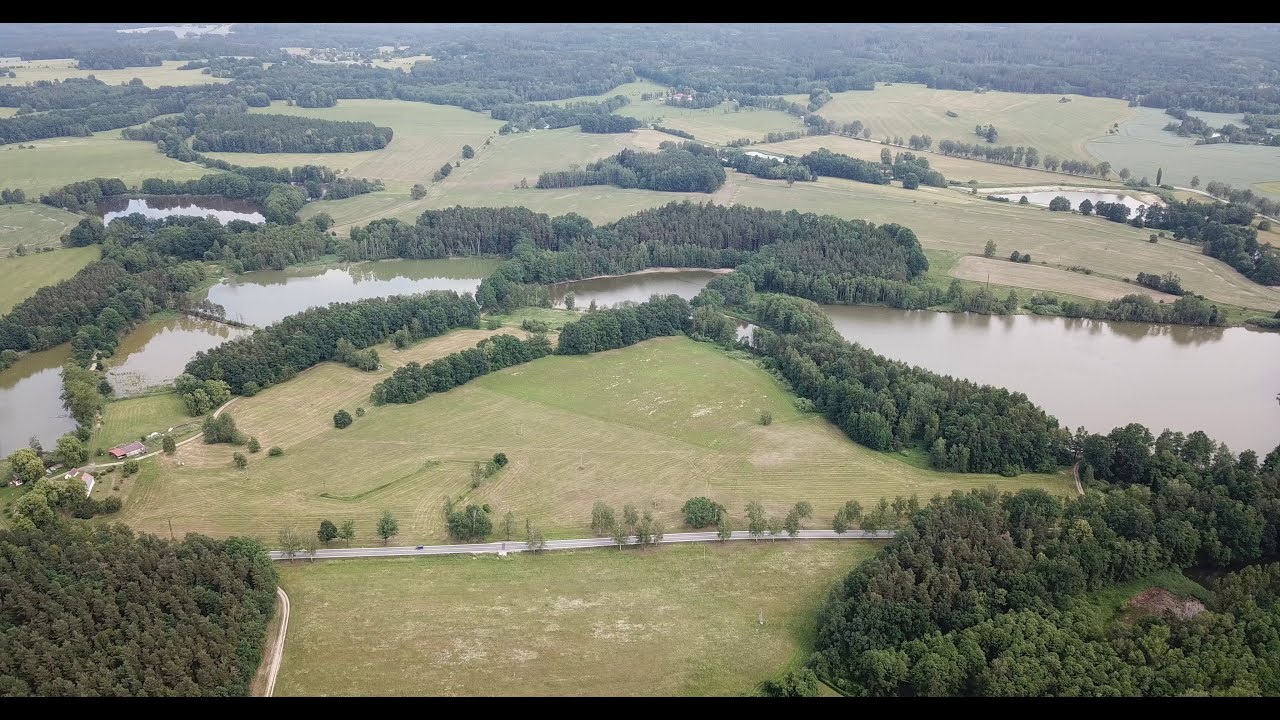The image presents a detailed aerial view captured from an elevation of approximately 100 to 200 feet, looking down at an angle over a mostly undeveloped landscape. Dominating the center of the image is a river flowing horizontally from left to right, bordered by clusters of darker green trees, especially concentrated in the middle area of the image. The surrounding landscape consists of gently rolling grasslands interspersed with isolated trees and smaller clusters. 

Noteworthy additions to the scene include several scattered ponds of varying sizes, creating the appearance of a series of water bodies, although they are separated by patches of trees, rendering the ponds distinct rather than part of a single connected river system.

A narrow road runs from left to right across the lower portion of the image, eventually disappearing behind a group of trees. There are a few signs of human habitation with occasional buildings visible, particularly in the bottom left quadrant of the image. Overall, the landscape is a patchwork of slightly hilly grasslands, random clusters of trees, distinct ponds, and a singular, central river, creating a rich tapestry of undeveloped natural beauty.